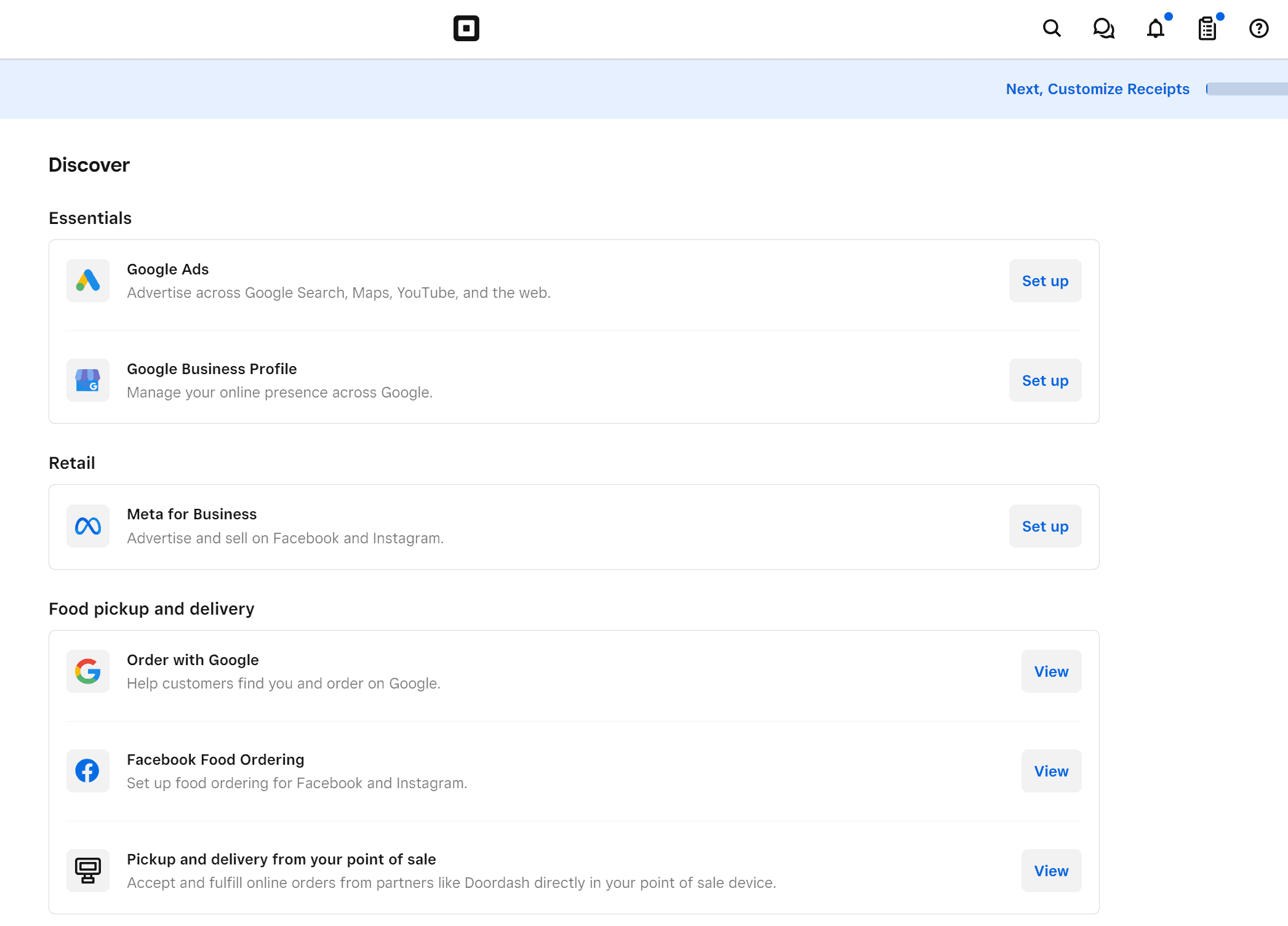The image is a large vertical screenshot, occupying most of the viewing space, set against a plain white background that seems to be borrowed from the computer screen. The focal point is a long, narrow blue rectangle that stretches down the height of the image. At the top of this blue rectangle is a black square with another black square inside it.

In the upper right-hand corner, still on the white background, are several small icons: a magnifying glass, a chat bubble, a bell, a calendar, and a question mark. Below these icons, within the blue rectangle, is the text "Customized Receipts" written in a darker blue, followed by a thin dividing line.

Shifting attention back to the left side of the image and below the blue rectangle, the word "Discover" is seen prominently, followed by bold black text "Essentials". Under the "Essentials" heading, there are sections detailing various services:

1. **Google Ads**: Accompanied by the Google Ads icon and further information about setting up Google Ads. To the right of this section, a setup button is available.
2. **Google Business Profile**: Includes details and an icon, with a setup button on the right.

Below is another bold heading titled "Retail":

1. **Meta for Business**: This section includes an image and information about advertising and selling on Facebook and Instagram, with a setup option.

Further down, under the heading "Food Pickup and Delivery" in bold black text:

1. **Google Food Ordering**: Featuring the Google icon, this allows users to order food.
2. **Facebook Food Ordering**: Highlighted with the Facebook icon, enables food ordering through Facebook.
3. **POS Food Pickup and Delivery**: Accompanied by a computer icon, describes ordering food directly from a point of sale system, with a "View" option available for each.

The layout is intuitive, offering setup and view options to the right of each section, facilitating easy interaction with the described services.